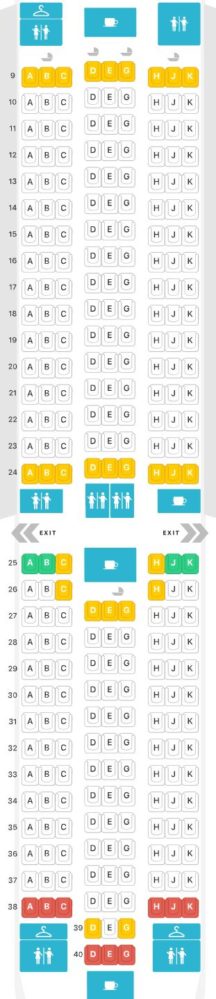The image depicts a detailed seating plan of an airplane, typically as seen on a computer or smartphone screen. The layout is presented vertically, with rows numbered from 9 to 40. Each row includes seats labeled A, B, C, D, E, G, H, J, and K. Different colors indicate various seat statuses or classes.

At the top, icons in teal depict amenities and exits. These include a teal box with a white hanger and two people icons, another box with a white cup resembling a cup of tea, and a third box with a person, a line, and another person.

Rows 9 and 24 have seats marked in yellow or yellow-orange, with adjacent teal icons. Rows 10 through 23 are entirely white. Rows 25 to 38 are more varied: 
- Row 25: Seats A and B are green, C is orange, D, E, G are white, H is orange, J and K are green.
- Row 26: Seat C is orange, D, E, G are white, H is orange.
- Row 27: Seats D, E, G are orange, others are white.
- Further rows mostly white, but Row 38 features red seats (A, B, C, H, J, K), Row 39 has orange seats (D, G), and Row 40 has red seats (D, E, G).

Exits are marked in the middle, with arrows pointing left and right. The teal icons appear periodically throughout the layout, indicating various in-flight amenities.